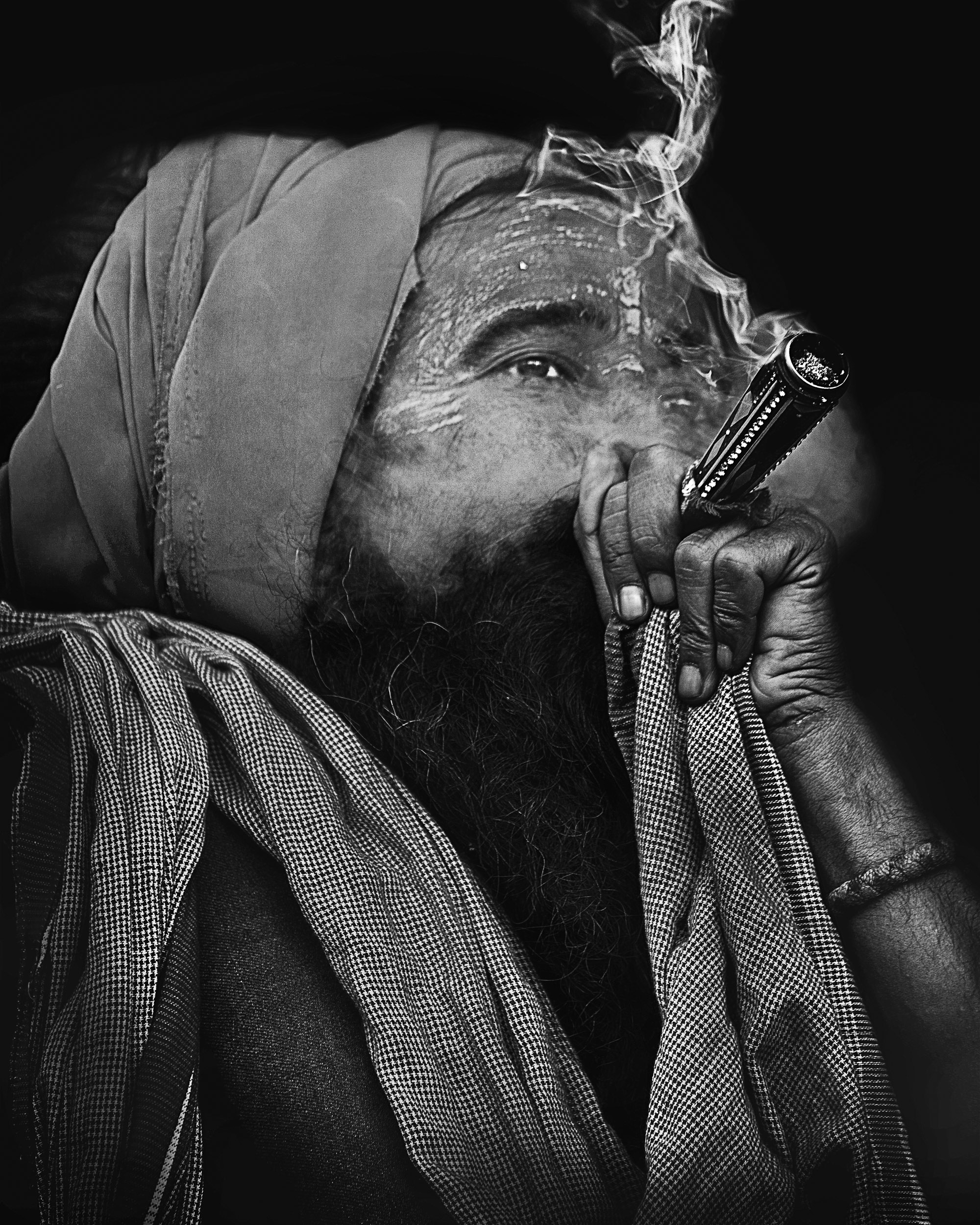This black and white photograph captures an older Indian man with a worn, wrinkled face, and a thick, slightly unkempt black beard. He is adorned with a head covering made of plain fabric and a checkered scarf that drapes over his shoulders. The man’s left hand, which has a bracelet on the wrist, is raised to his mouth, holding an ornate pipe that seems to be adorned with designs and possibly gems. A stream of intricate, swirling smoke from the pipe envelops his face, obscuring his mouth and one of his dark, distant-looking eyes, while accentuating the other. The background of the image fades into darkness, enhancing the focused, contemplative expression in his visible eye as he stares off to the right. Despite the obscurity of some details due to the smoke and shadow, the photograph richly portrays the man's somber and reflective demeanor.